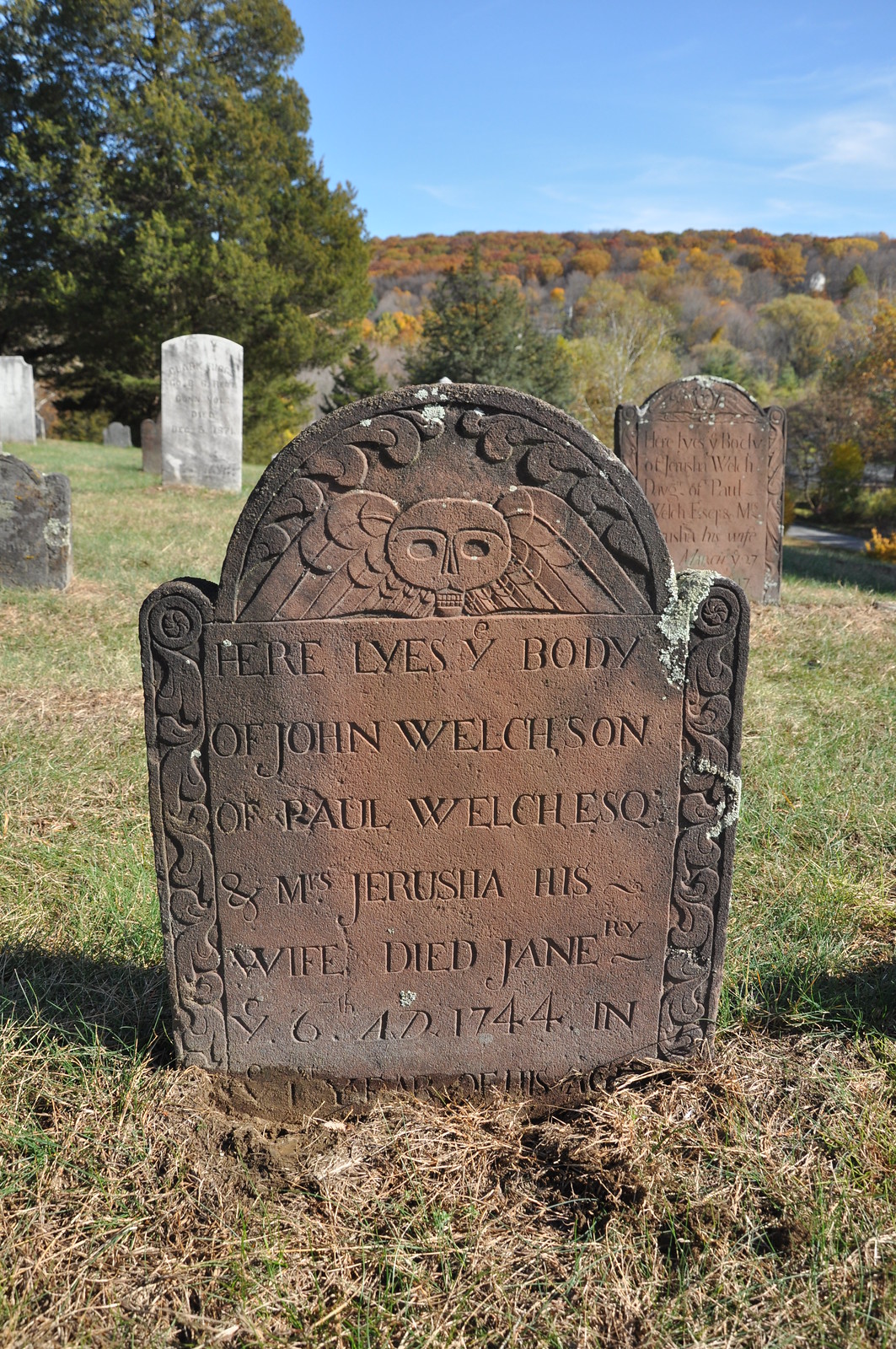The photograph depicts an old cemetery bathed in mixed shades of green and brown grass with patches of weathered terrain. In the center, a prominent tombstone stands tall, rectangular with a semi-circular top, made of stone that has darkened in places over time, giving it a brownish hue. The tombstone, worn and weathered, bears intricate carvings including a skull and winged designs flanking its sides. The engraved text reads: "Here lies the body of John Welchson, son of Paul Welchson and Mrs. Jerusha, his wife, died June 6, A.D. 1744, I.N." This historic marker, partially obscured by encroaching weeds, symbolizes the passage of time. Surrounding it, other headstones dot the grassy field, while a backdrop of many trees frames the blue sky above, completing the serene yet somber scene.